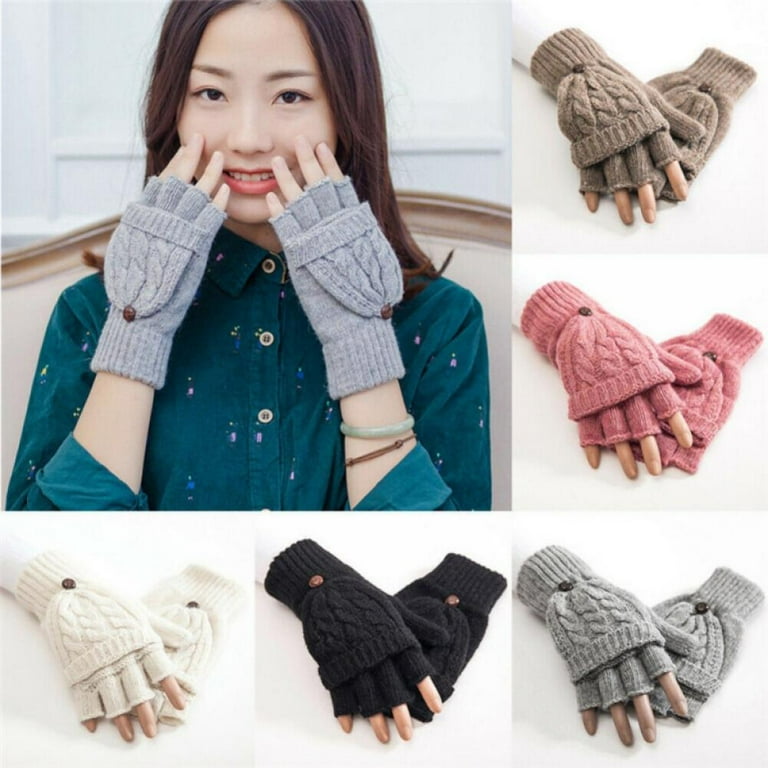The image features a 3x3 grid primarily themed around fingerless gloves. The top-left section, a merged larger image, showcases an Asian woman from the chest up, smiling and holding her fingers to her chin. She wears dark greenish-blue buttoned shirt and a pair of gray fingerless gloves made from a knit material. The gloves extend slightly past her wrists, and feature flaps that resemble mini beanie hats pulled back to expose the fingers. The gloves also have small wooden circle embellishments near the finger openings. Notably, the woman accessorizes with a jade bracelet, another thin brown bracelet, and a turquoise blue bubble wrap. The remaining five images in the grid depict the same style of gloves in various colors—tannish brown, muted mauve pink, gray, black, and white—each modeled on a right hand with the left glove displayed underneath. Each glove, identical in design, features the finger-covering flap pulled back, revealing the fingers.